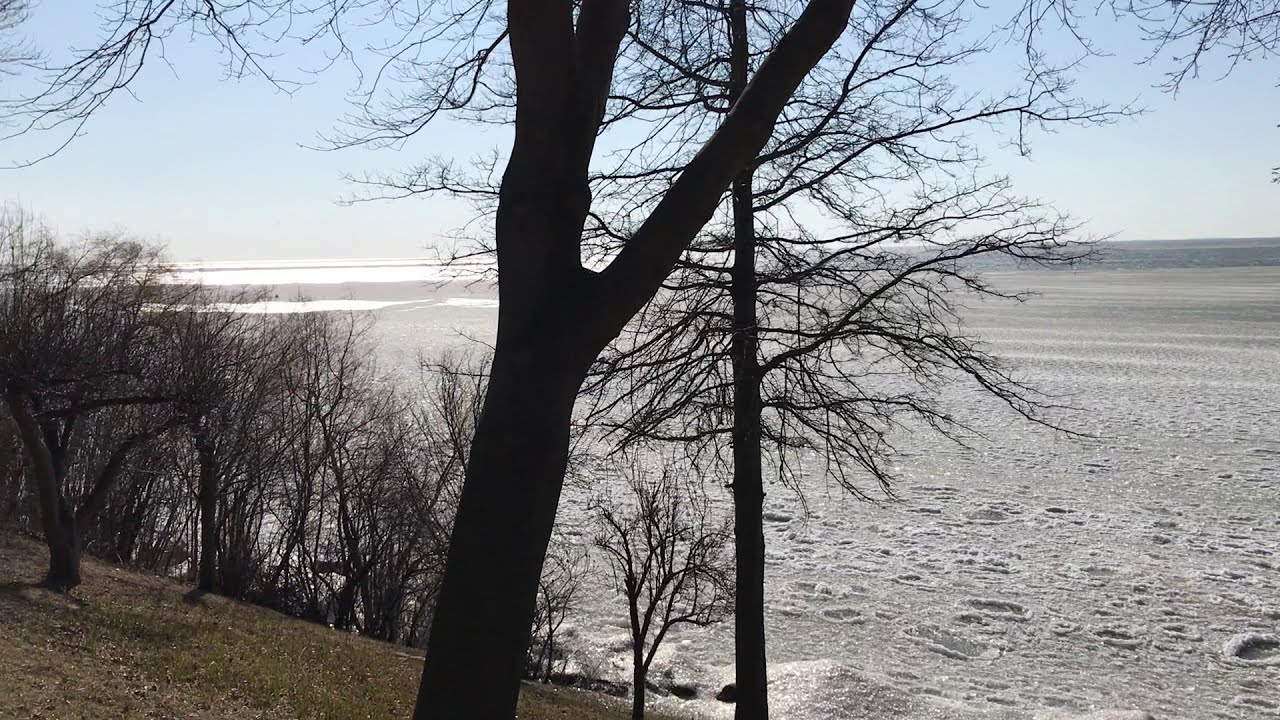In the heart of winter, this outdoor image showcases a frozen lake sprawling far into the horizon. Central to the scene stands the striking silhouette of a leafless tree, its trunk angling gracefully before splitting into three prominent branches. To the right, a sloped grassy hill, interspersed with dirt patches, gently descends towards the icy expanse. Dotted along this hill are sparse, twig-like trees devoid of leaves. The frozen lake's surface is marked by countless craters, divots, and pockets of water, creating a textured mosaic. In the top left, sunlight glistens, casting a reflective light on the ice, while the pale blue sky without clouds stretches across the upper third of the image. Along the horizon, additional flat land outlines the vast body of water, which might be part of one of the great lakes, extending the frozen scenery into the distance. The serene scene is further enriched by the visible glare from the sun, illuminating the top left and hinting at the midday light.